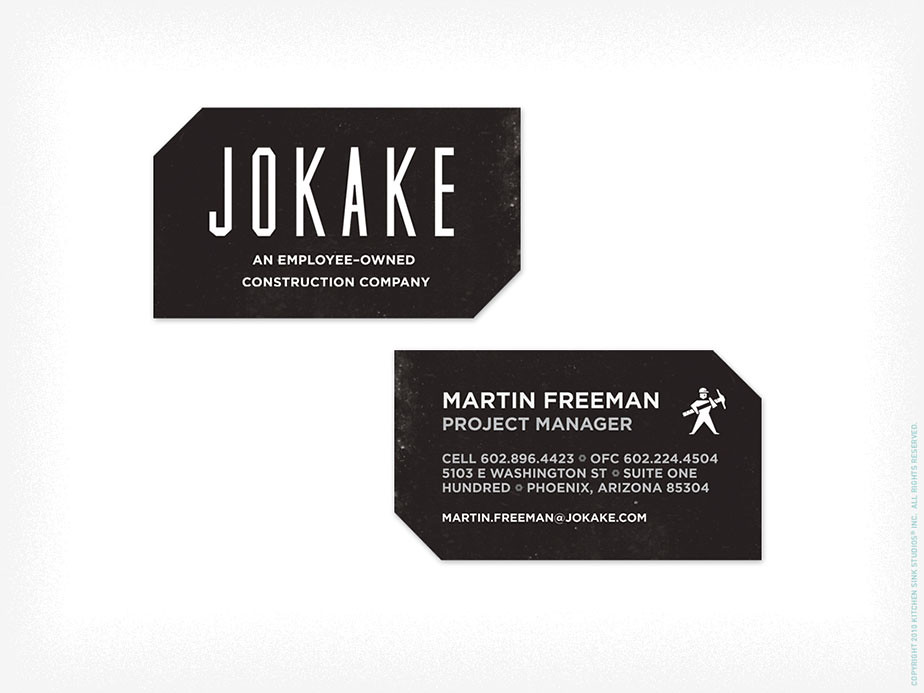The image presents two business card-like drawings on a light blue background, with a white border. The cards have a visually distinct appearance due to their unique corner cuts. The top card features the text "JOKAKE" prominently in bold, white capital letters. Beneath this, in smaller white font, it states "an employee-owned construction company." The bottom card, slightly to the right, also has a black background. It reads "Martin Freeman, Project Manager" at the top and includes a small, cartoonish icon of a man in a helmet holding a large pickaxe, positioned to the right. Below this, the card provides Martin's contact information: Cell: 602-896-4423, Office: 602-224-4504, Address: 5103 East Washington Street, Suite 100, Phoenix, Arizona, 85304, and his email, MartinFreeman@jokake.com.